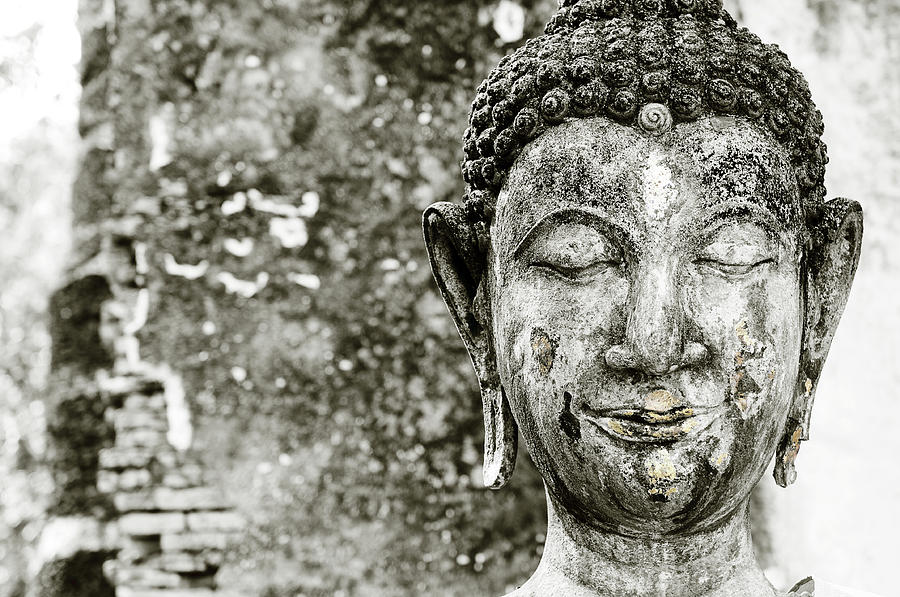The image is a black-and-white photograph of a weathered Buddha statue, featuring the head and part of the upper body. The statue shows the serene face of a male Buddha with eyes closed and a half-smile. The nose is long, and the large ears reflect the Buddha's story as a wealthy man whose earrings stretched his earlobes. The Buddha's head is adorned with a dark, studded headpiece made of small circles arranged in a swirling pattern, indicative of traditional depictions. However, the headpiece is truncated as the top is cut off by the photo's frame.

The statue bears evidence of age and wear, with noticeable gouges and chipped areas, especially on the lower part of the face. The overall color of the statue is a mix of gray and black, with dirt and mud adding to its worn appearance. The forehead has visible gray markings, contributing to its aged look. 

In the background, a large tree trunk can be seen, suggesting the statue is situated outdoors. The backdrop further includes a worn gray and black wall with numerous white scratches, reinforcing the sense of historical decay. There is no text in the image, and the setting underscores the timeless and tranquil essence of the Buddha amidst nature and time.